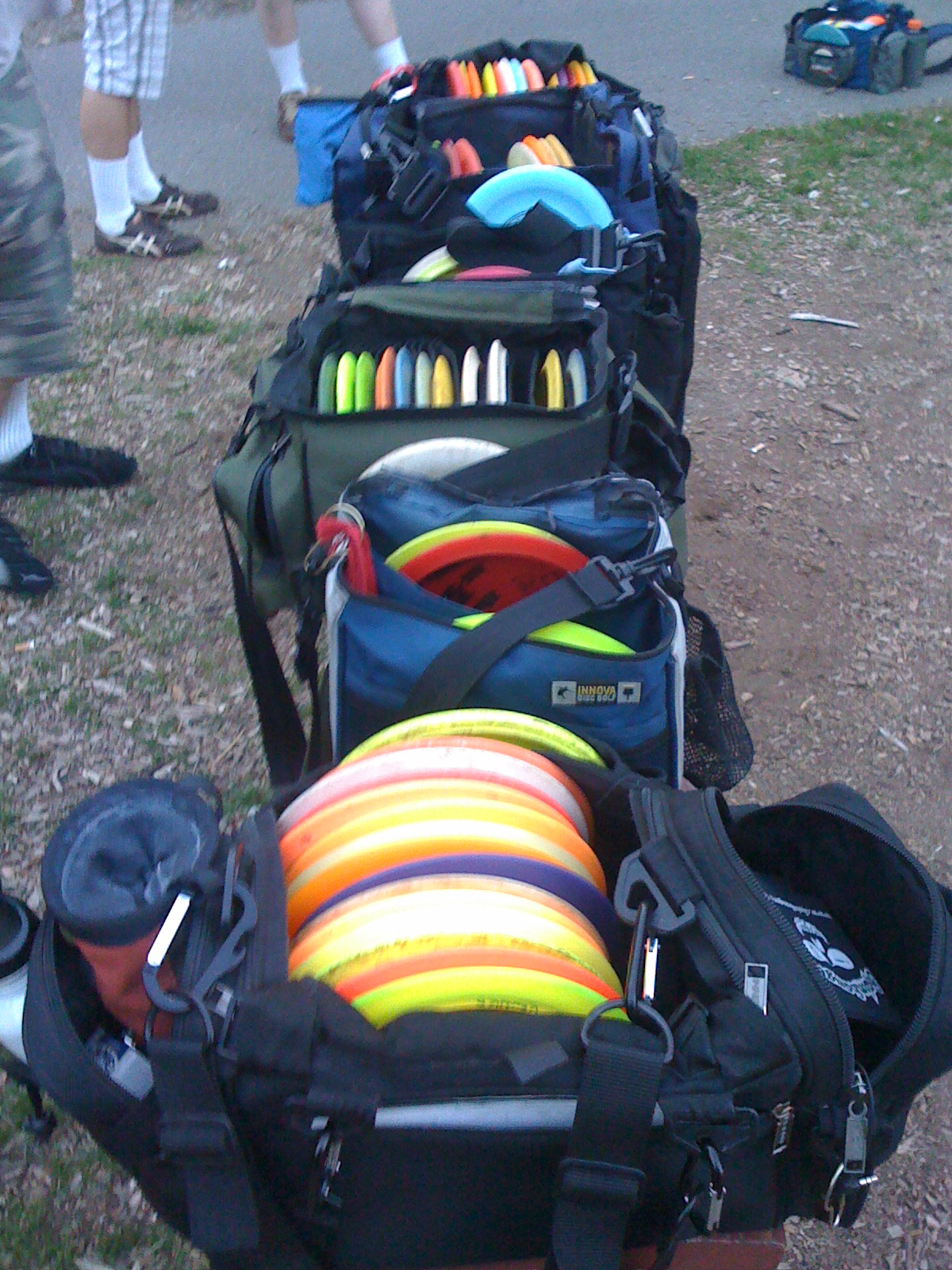In this slightly blurry and dark amateur photograph taken from above, we see a scene set outdoors on a predominantly dirt-covered field with patches of grass. The main focus is on six black bags, which appear to be specialized carriers, possibly for a frisbee or disc golf event. Each bag is packed with a multitude of colorful frisbees—red, blue, white, yellow, pink, and green—holding them securely within zippers and side pockets, some of which are designated for holding drinks. The arrangement of the bags forms a line stretching across the image, suggesting an organized setup. In the upper right corner, a concrete pathway intersects the dirt and grass, with yet another frisbee-filled bag resting nearby. The lower left of the frame shows the partial lower bodies of three individuals, identifiable only by their legs and feet; they are sporting white socks and dark shoes, wearing shorts that expose their calves. This image, captured during the day, offers a glimpse into what might be preparations for a frisbee competition or casual ultimate frisbee games.